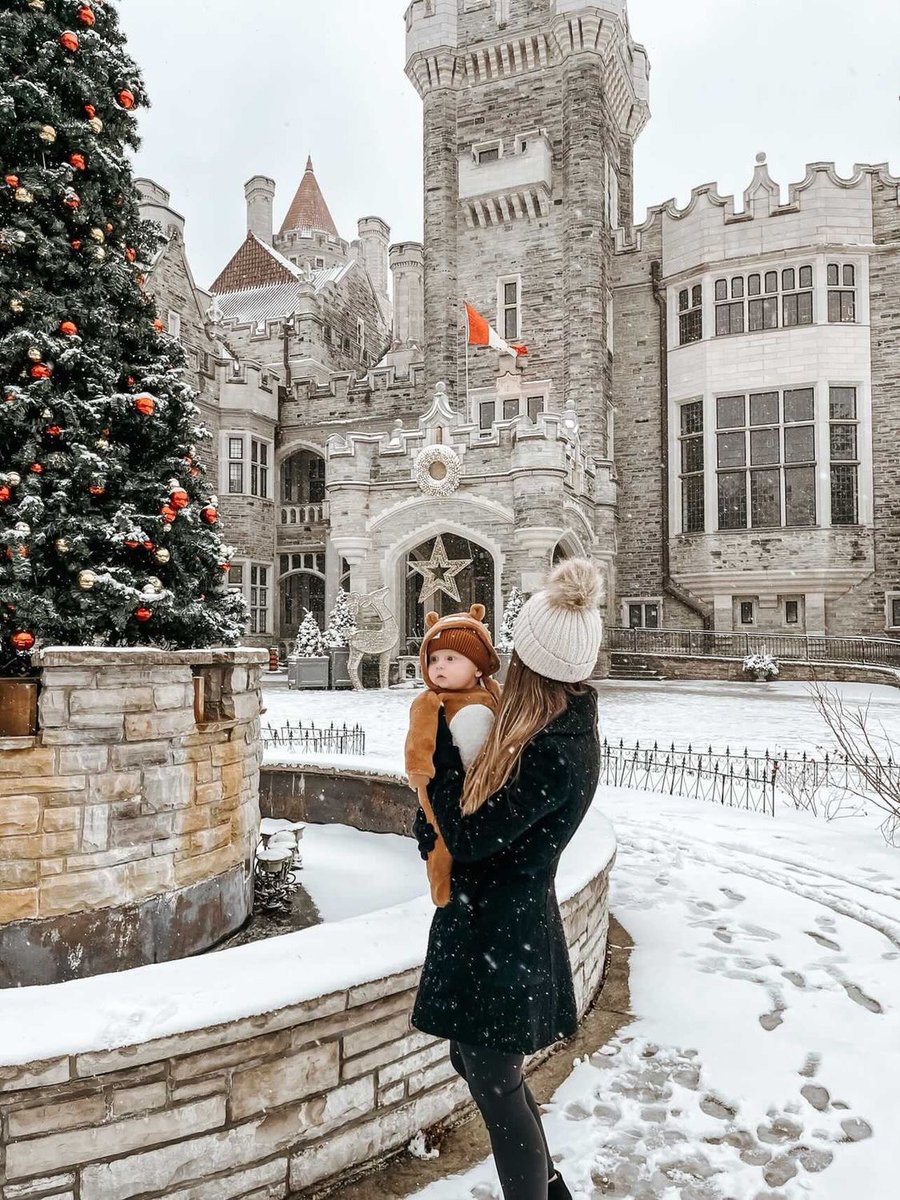In this outdoor photograph, a woman with long blonde hair stands in the middle of a snow-covered ground, holding a baby. Captured from the side, she looks to her right at a large, ancient-looking grey building adorned with multiple windows and a flag atop it. The woman is dressed in a dark green or black coat, grey pants or leggings, and a cream or white pom-pom hat. She cradles her baby, who is bundled up in a tan or brown costume with ear details on the hood. To the left of the woman is a partially visible dark green Christmas tree decorated with red and white ornaments. The tree is situated on a platform surrounded by a brick barrier that reaches knee-height. The sky overhead is light blue and clear, adding to the wintry atmosphere.